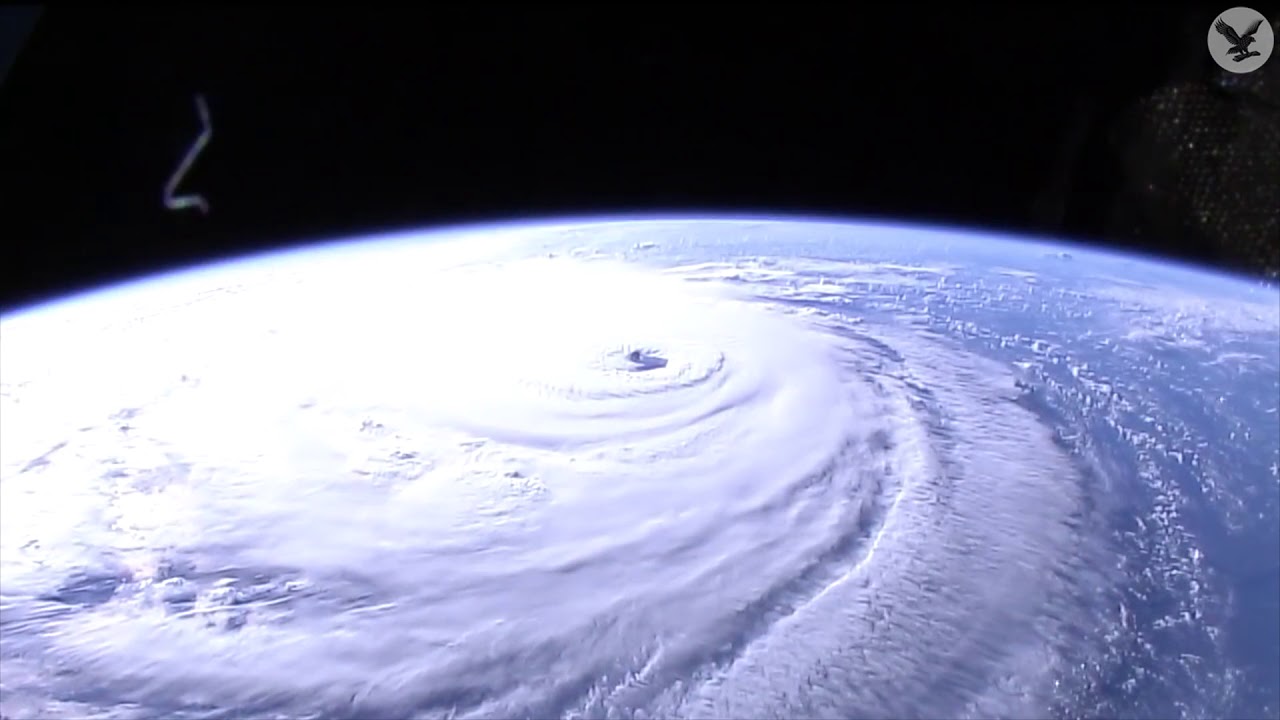The image captures a breathtaking view from space, highlighting the juxtaposition of the vastness of the cosmos and the dynamic processes on Earth. The backdrop is the deep blackness of space, punctuated by a scattering of small, sparkling stars in the top right-hand corner. Dominating the bottom portion of the frame is the vibrant blue curvature of Earth, suggesting the presence of oceans teeming with life.

At the center of the image, a massive hurricane takes form, its imposing presence manifesting as a giant, swirling mass of thick, white clouds. The clouds spiral tightly, resembling a colossal whirlpool, with striking detail and intensity. The eye of the hurricane stands out as a small, dark void at the center of this atmospheric vortex, reminiscent of a typhoon or tornado, highlighting the fierce energy contained within.

Surrounding the hurricane, the lighter blue hues of the ocean add to the complexity of the scene, contrasting dramatically with the deep blue of the Earth’s curvature. In the top left-hand corner of the image, a mysterious bright string-like reflection appears to dangle, adding an enigmatic touch to the composition, its nature unclear yet intriguing.

Overall, the image offers a powerful perspective on the stark beauty and raw force of nature as observed from the serenity of space.